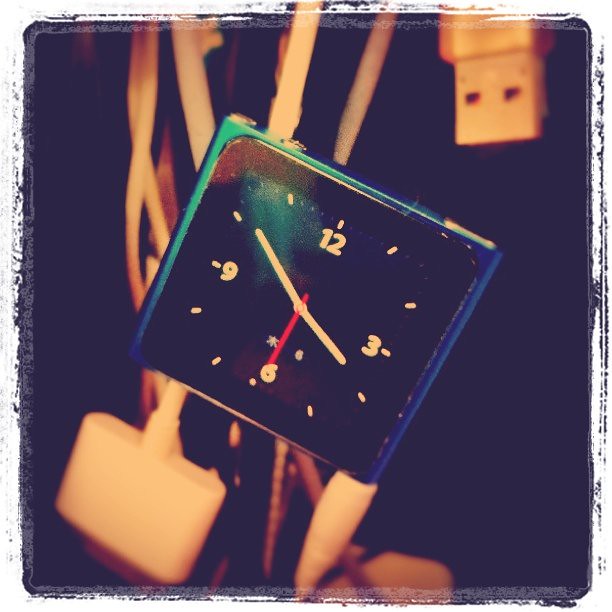The image depicts a small, square electronic device, likely an iPod, featuring a bluish metallic, shiny finish. Prominently displayed on its screen is a clock interface. The clock displays the numbers 3, 6, 9, and 12 with two white dashes marking each interval between the numbers. Notably, there is a small star symbol above the number 6, with another minuscule number 6 positioned just above the star. The clock's hands are positioned as follows: the small hand points at 4, the large hand at 10, and the second hand at 6, the latter being distinguished by its red color, while the other hands are white. Connected to the device is a pair of headphones and a white USB cable that dangles behind it. The border of the image appears to be deteriorated, adding a distressed aesthetic to the photograph.